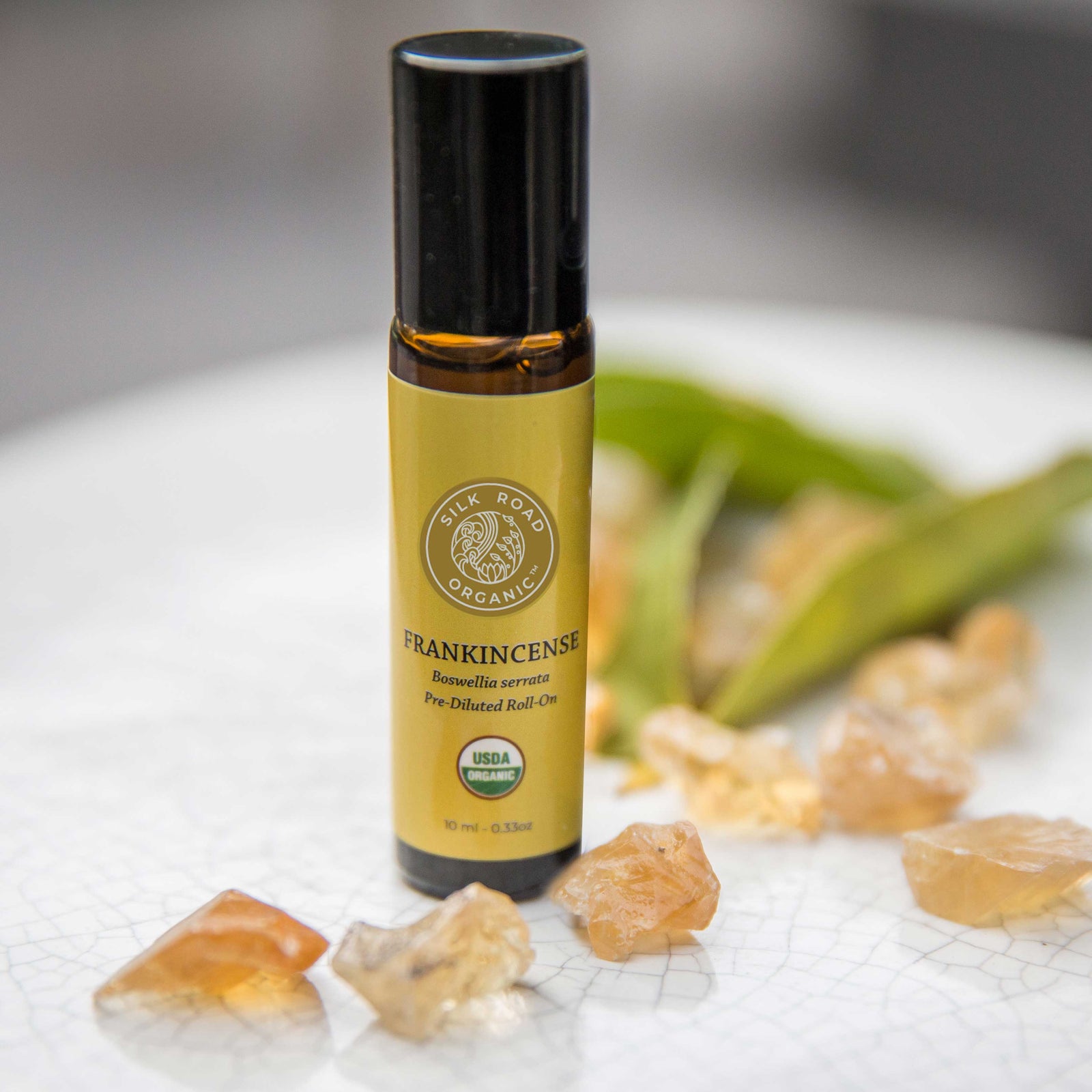The close-up image is a detailed product photograph of an amber-colored glass bottle labeled "Silk Road Organic Frankincense," prominently displayed on a white, crackled plate. The bottle has a sleek black plastic cap and features a circular gold label with white text, including a gold logo that reads "Silk Road Organic" and the word "frankincense" beneath it. Below the logo are several lines in a foreign language, as well as a round USDA Organic symbol. Surrounding the bottle are scattered golden amber-colored rocks and crystals, adding a tactile element to the composition. To the right, there are a few out-of-focus green leaves, possibly celery or green beans, providing a natural touch to the scene. The photograph is a square format, emphasizing the aesthetic and commercial appeal of the frankincense product, capturing fine details to convey a sense of luxury and organic purity.